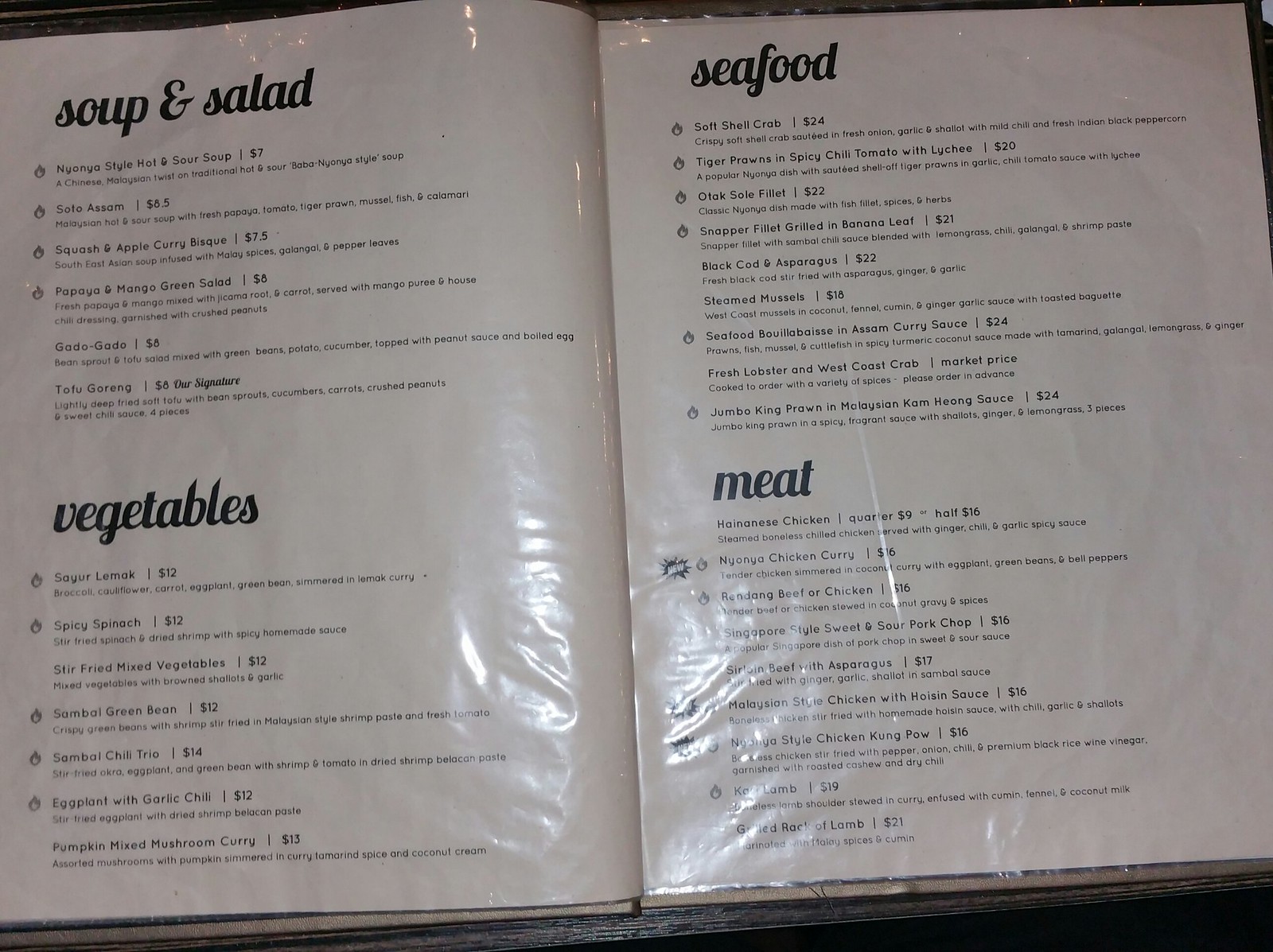The image features a restaurant menu, displayed open to reveal its two full pages. The menu is set against a pristine white background with sleek black printing that is covered with a glossy, reflective material, possibly cellophane. There is noticeable gathering of this material at the bottom edges. 

On the left-hand page, the menu is divided into distinct sections. At the top, the heading reads "Soup and Salad," followed by a detailed list of items under this category along with their respective descriptions and prices. Below this section is another heading labeled "Vegetables," which similarly enumerates the available vegetable dishes and their prices.

The right-hand page is organized into two primary sections. At the top, "Seafood" is boldly printed, introducing an assortment of seafood dishes. Certain items are marked with small fire icons, indicating their spiciness. Following the seafood section is the "Meat" category, listing various meat-based dishes along with their descriptions and prices.